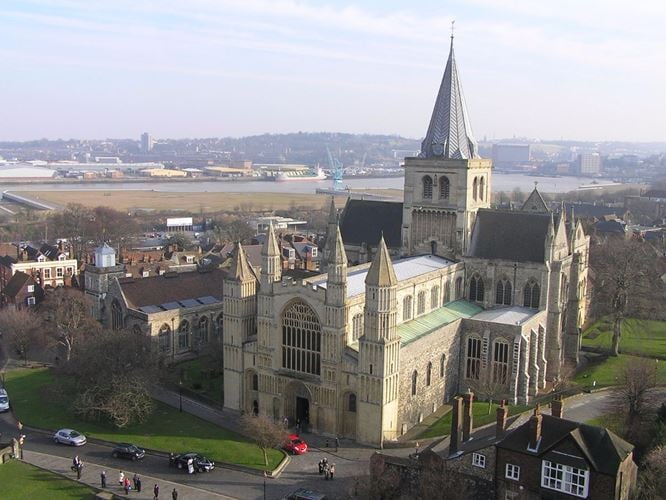This is an aerial photograph capturing a grand, beige stone church set amidst a well-maintained, bright green lawn. The church stands impressively tall with multiple spires, the most prominent being a large main spire at the back, which is the tallest and crowned with a small antenna or cross. The front facade features four spires and several entranceways, including a significant main archway. The roof displays a striking pattern with sections of gray, white, and green. The scene is under a hazy sky dotted with wispy white clouds that allow glimpses of blue. The sunlight, unseen in the photo, appears to be coming from the right. Surrounding the church are manicured grassy areas and a driveway where cars are parked, with neatly dressed people coming and going. In the backdrop, a large river or possibly a lake meanders through rolling hills and an urban landscape, adding to the majestic and serene ambiance of the scene.